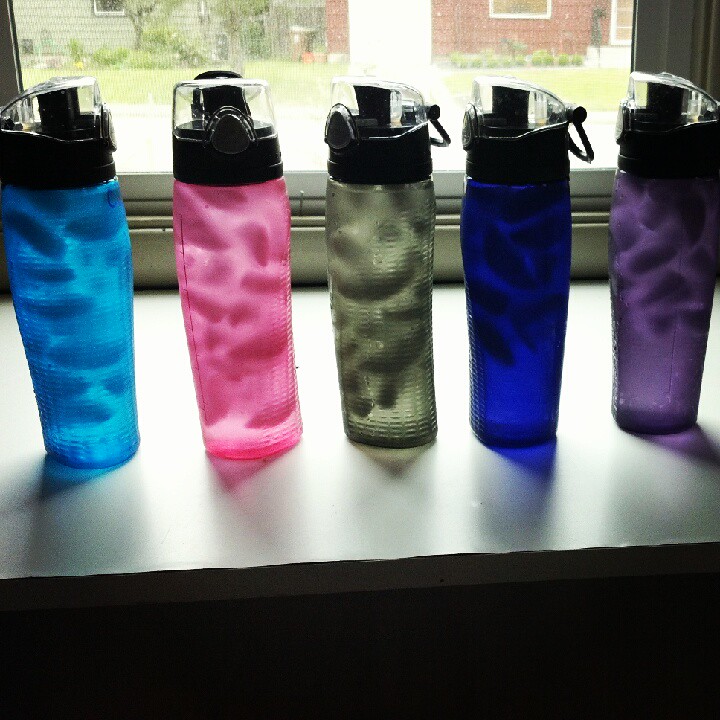This photograph captures five water bottles meticulously lined up on what seems to be a shiny, vinyl or laminated kitchen countertop. Each bottle is of the same size and design, featuring a distinctive black cap with a white plastic snap-over cover that includes a loop for easy hanging. The bottles are filled with clear water and ice cubes, likely from an ice maker. They are transparent, and their colors transition from left to right as follows: light blue, pink, gray, dark blue, and purple.

The window behind the bottles bathes the scene in natural light and showcases an outdoor view. Through the window’s metal frame and possible screen, you can see a well-manicured lawn and two houses in the distance. One house features red wood or paneling, and the other has sections that appear either white or green. This setting, combined with the neatly arranged, colorful bottles, creates a visually appealing and serene image of daily life.